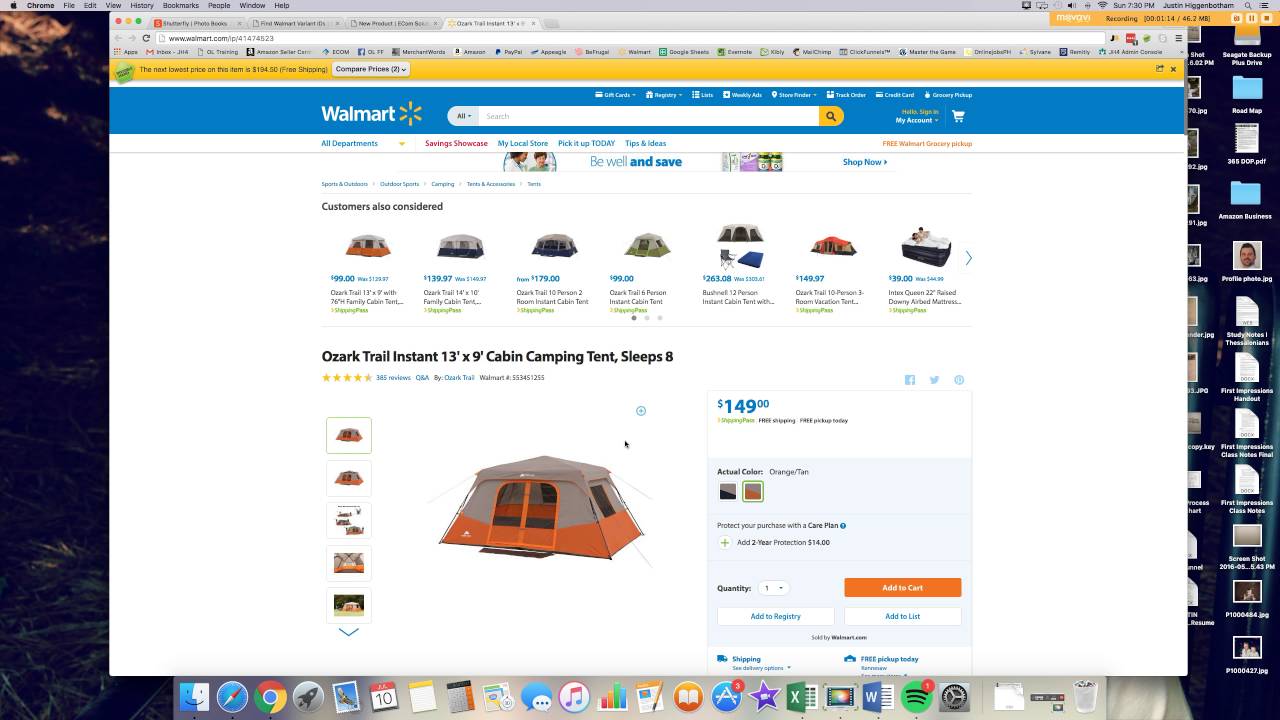The image depicts a computer screen displaying a webpage from the Walmart website. The webpage takes up about 80% of the screen and features a search bar, a shopping cart icon, and a user account option. The interface showcases the "All Departments" section highlighted in blue. Below, there's a section titled "Customers also considered," displaying various tents. There are seven tents in total, with the last one resembling a bed.

The highlighted product is the "Ozark Trail Instant 13-foot by 9-foot Cabin Camping Tent," which can accommodate up to eight people. The tent is priced at $149, shown in blue text. The image displays two color variants of the tent: one in orange and beige (orange at the bottom) and the other in black and beige (black at the bottom). An orange "Add to Cart" button is prominently featured on the page.